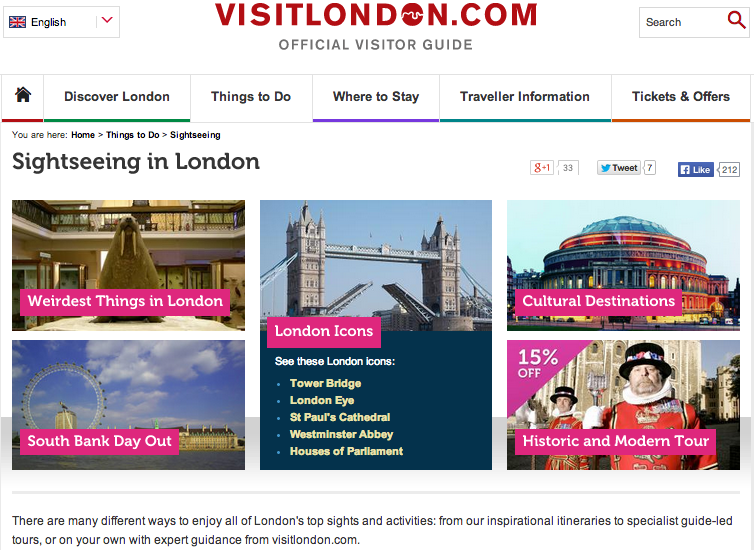The image is a screenshot from a website, likely displayed on a desktop or laptop screen, showcasing the homepage of visitlondon.com. At the top center of the page, the website title "visitlondon.com" is prominently displayed in bold red block letters. The letter "O" in "London" is styled as a solid red circle with jagged borders, resembling the outline of a geopolitical boundary. Just below the title, the tagline "Official Visitor Guide" is written in grey text.

To the right of this tagline, there is a search bar. Beneath this header section, there are six navigational tabs arranged horizontally: Home, Discover London, Things to Do, Where to Stay, Traveler Information, and Tickets and Offers. Each tab is underlined with a distinct color: red, green, purple, green (or possibly blue), and orange. Interestingly, the highlighted tab, "Things to Do," lacks an underline color, which is unconventional as the highlighted tab typically has a color for emphasis.

Further down, the section titled "Sightseeing in London" includes several images accompanied by pink boxes with white text captions such as "Weirdest Things in London," "London Icons," "South Bank," and "Day Out." This detailed layout underscores that the website is designed as a tourist resource for exploring London.